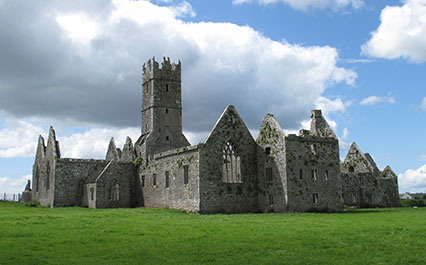This detailed outdoor daytime photograph showcases the ruins of an old Gothic-style stone church or castle. Dominating the scene is a towering rectangular spire that rises above a series of low-lying stone buildings, which collectively appear weathered and worn. The structures are made from gray stone, assembled in a way that resembles a tapestry of rocks. Notable architectural elements include several gabled roofs missing their coverings, suggesting possible flat roofs beneath or the remnants of former roofs.

Surrounding the central tower are four distinct buildings. To the left, a structure with gabled ends but no visible roofing may indicate a flat roof or roofless element. Next, a slightly taller square-shaped building with four windows and a prominent archway. Adjacent to it is another similar building, characterized by its gabled ends and rectangular silhouette. At the bottom of the image, additional low-lying structures continue the theme of gabled roofs.

The foreground is a lush, vibrant green field that contrasts sharply with the gray stone constructions. The serene blue sky above is punctuated by a mix of fluffy white clouds and a larger, slightly gray cloud extending from the left to the middle. The picturesque scene captures the beauty and historical intrigue of an ancient, partially preserved architectural marvel, offering a glimpse into its storied past through its enduring stone walls and the verdant surroundings.